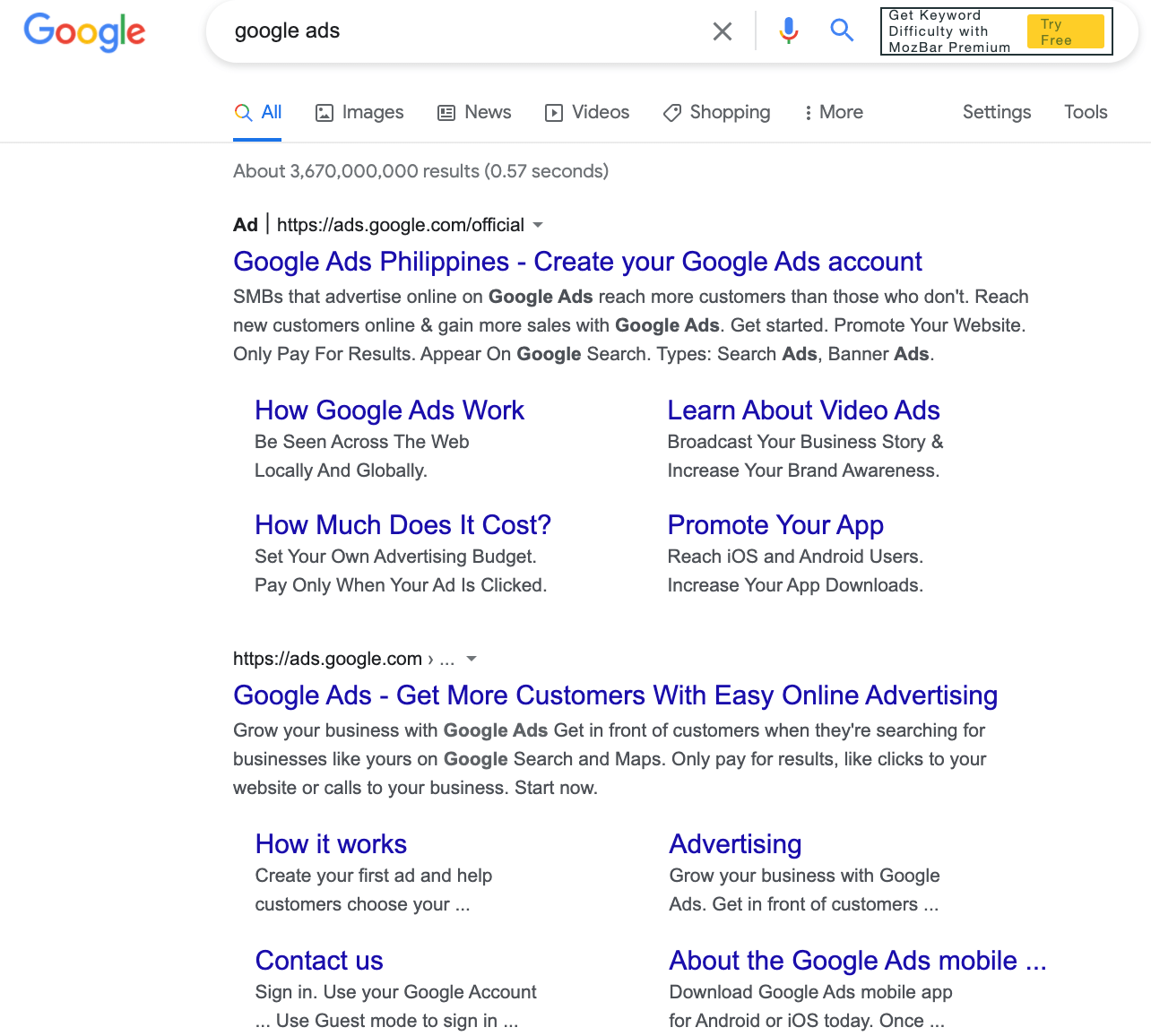In this photographic image, the Google logo, featuring the iconic blue "G," red "o," yellow "o," blue "g," green "l," and red "e," is prominently displayed in the top left corner. Below the logo is a search bar indicating a query for "Google Ads," flanked by an 'X' on the left and a microphone icon on the right.

The search results page reveals a highlighted box at the top offering a trial for "MozBar Premium" to obtain keyword difficulty metrics. Below this, the search results are segmented into various categories: "All," "Images," "News," "Videos," "Shopping," and "More," each accompanied by a microphone icon.

The display shows an impressive 3,670,000,000 results delivered in just 0.57 seconds. The first few hyperlinked results include:
- "Google Ads Philippines - Create your Google Ads account"
- "How Google Ads works"
- "Learn about video ads"
- "Promote your app"
- "How much does it cost"

In addition, there are links to:
- "Get more customers with easy online advertising"
- "How it works"
- "Contact us"
- "Advertising"
- "About Google Ads mobile"

The page layout also includes options to access "Settings" and "Tools" for further refinement or customization of the search experience.